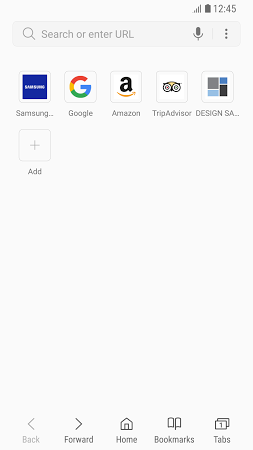This image displays a screenshot of a smartphone's home screen, populated with a variety of app icons. At the very top of the screen, the smartphone status bar is visible, showcasing standard indicators: a signal strength icon, a battery icon, and a clock, confirming the device is operational and connected.

Just below this status bar is a search bar with a text placeholder that reads "Search or enter URL." The presence of a microphone icon within this bar suggests the capability for voice-activated searches, enhancing user convenience.

The screen features a selection of prominent app icons. Among them is the Samsung app, identifiable by its blue and white logo. Adjacent to it is the Google app, marked by its distinctive multicolored capital "G." The Amazon app is also present, featuring a lowercase "a" with an arrow resembling a smile curving beneath it. Another recognizable icon belongs to TripAdvisor, which displays a stylized owl's face.

Additionally, there is an app with the label "Design Essay," although the text is truncated and the full name is not entirely visible. This icon consists of a composite of smaller squares and rectangles, in colors of blue, gray, and black. Each app icon is precisely detailed, providing a clear look at the organization of this smartphone's home screen.